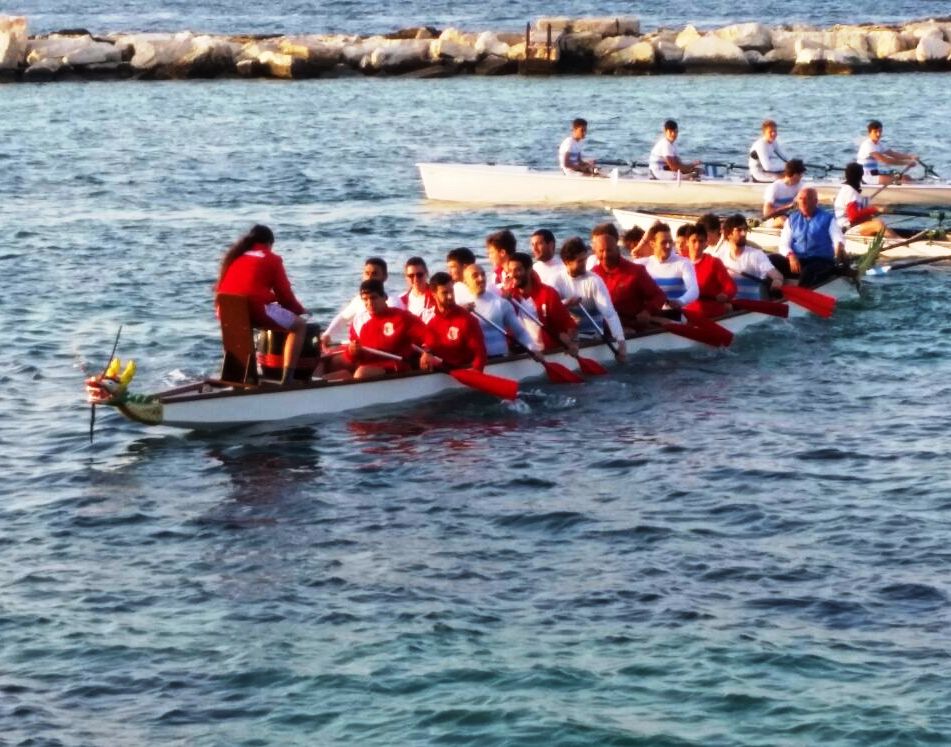The image shows three rowing teams on a body of water bordered by a stone wall separating it from another body of water. The largest boat in the foreground, a canoe-like vessel, contains around 16 to 20 people, predominantly dressed in red and white shirts. A person in a red jacket is standing at the bow, likely a coach, while a man in a blue vest stands at the stern. Behind this boat is a smaller canoe with two visible rowers, heading off to the left. Furthest in the background, a white rowing boat with four rowers is visible, moving to the right. The scene captures the vibrant activity on the water with a rocky shoreline in the backdrop, emphasizing a dynamic and lively rowing event.